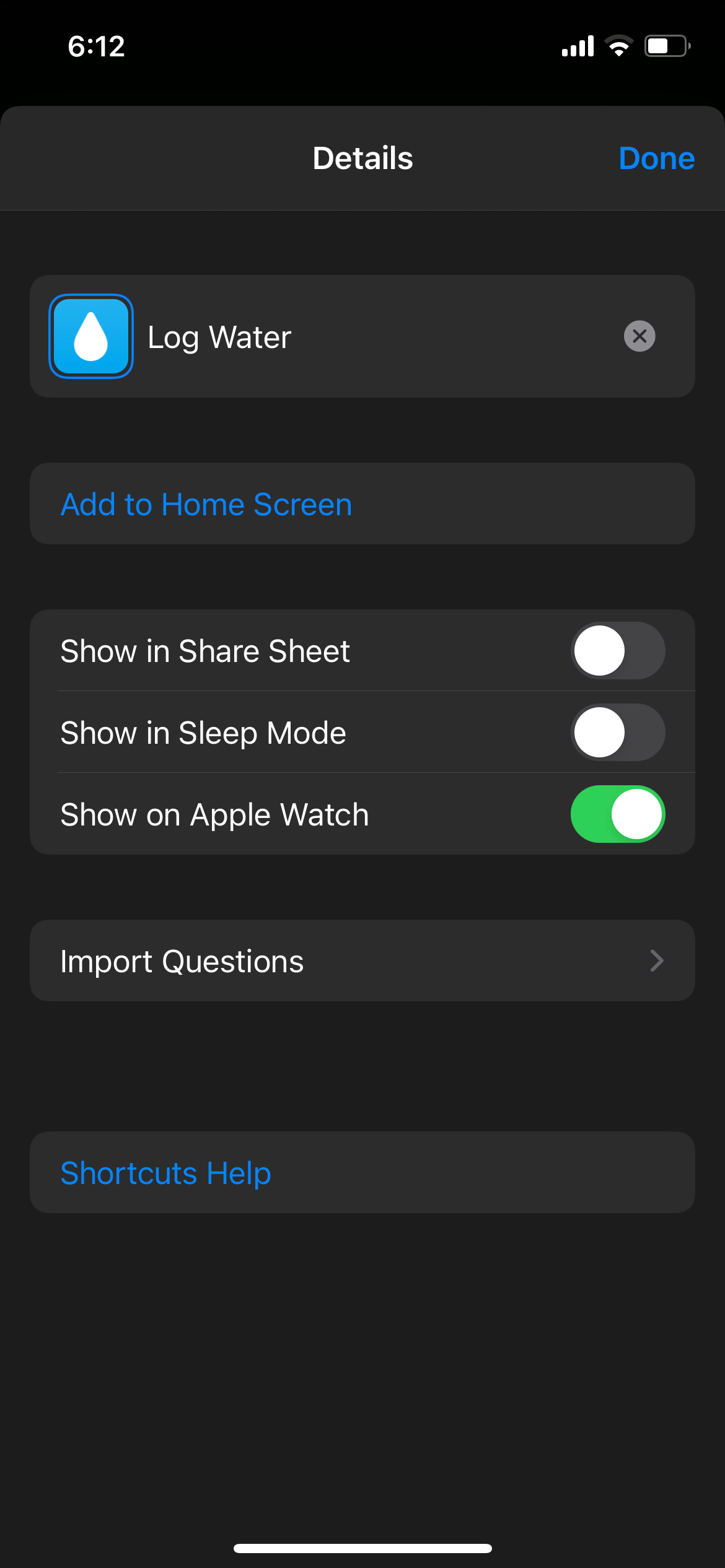Screenshot of a mobile phone settings screen—likely an Apple automation app—displayed on a black background. The status bar at the top of the screen shows the time as 6:12 in the upper left-hand corner, and in the upper right-hand corner, indicators show four bars of mobile signal strength, two bars of Wi-Fi, and a half-full battery icon without a percentage.

Below the status bar is a lighter black rectangle. In the center of this rectangle, white text provides details, while “Done” appears on the far right in blue. 

A third of the way down the screen, a white horizontal bar divides the content. Beneath this are several more rectangles. The first rectangle has "Log Water" written in white text on the left with a blue square icon featuring a white water droplet next to it, along with an "X" to close it.

Following that are additional rectangles:
- One with blue text reading "At Home Screen"
- Another stating "Show in Shares Sheet" (not selected), "Show in Sleep Mode" (not selected), and "Show on Apple Watch" (selected with a green slider)

Below these options, there are more sections:
- An "Import Questions" option marked with a forward arrow
- Finally, a rectangle with blue text on the left side reading "Shortcuts Helps"

The screen appears to be oriented around managing or configuring a specific app, possibly related to logging water intake based on the context clues.